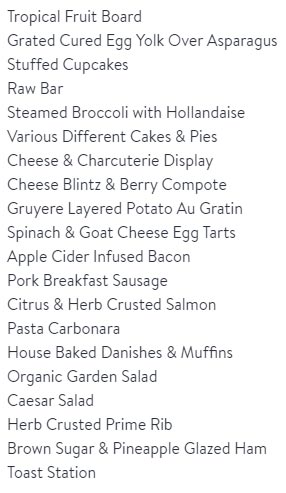The image features a detailed vertical list of various gourmet foods set against a white background, with no border framing the text. The text itself is presented in a light gray color, utilizing a mix of capital and lowercase letters for each item. The list includes:

1. Tropical Fruit Board
2. Grated Cured Egg Yolk Over Asparagus
3. Stuffed Cupcakes
4. Raw Bar
5. Steamed Broccoli with Hollandaise
6. Various Cakes and Pies
7. Cheese and Charcuterie Display
8. Cheese Blintz with Berry Compote
9. Gruyere Layered Potato Au Gratin
10. Spinach and Goat Cheese Egg Tarts
11. Apple Cider Infused Bacon
12. Pork Breakfast Sausage
13. Citrus and Herb Crusted Salmon
14. Pasta Carbonara
15. House Baked Danishes and Muffins
16. Organic Garden Salad
17. Caesar Salad
18. Herb Crusted Prime Rib
19. Brown Sugar and Pineapple Glazed Ham
20. Toast Station

The arrangement and variety of items suggest this could be a menu for a buffet, a special gathering such as a wedding, or a restaurant. Each food item is listed plainly and elegantly without additional visuals or border decorations, emphasizing the simplicity and straightforwardness of the menu presentation.